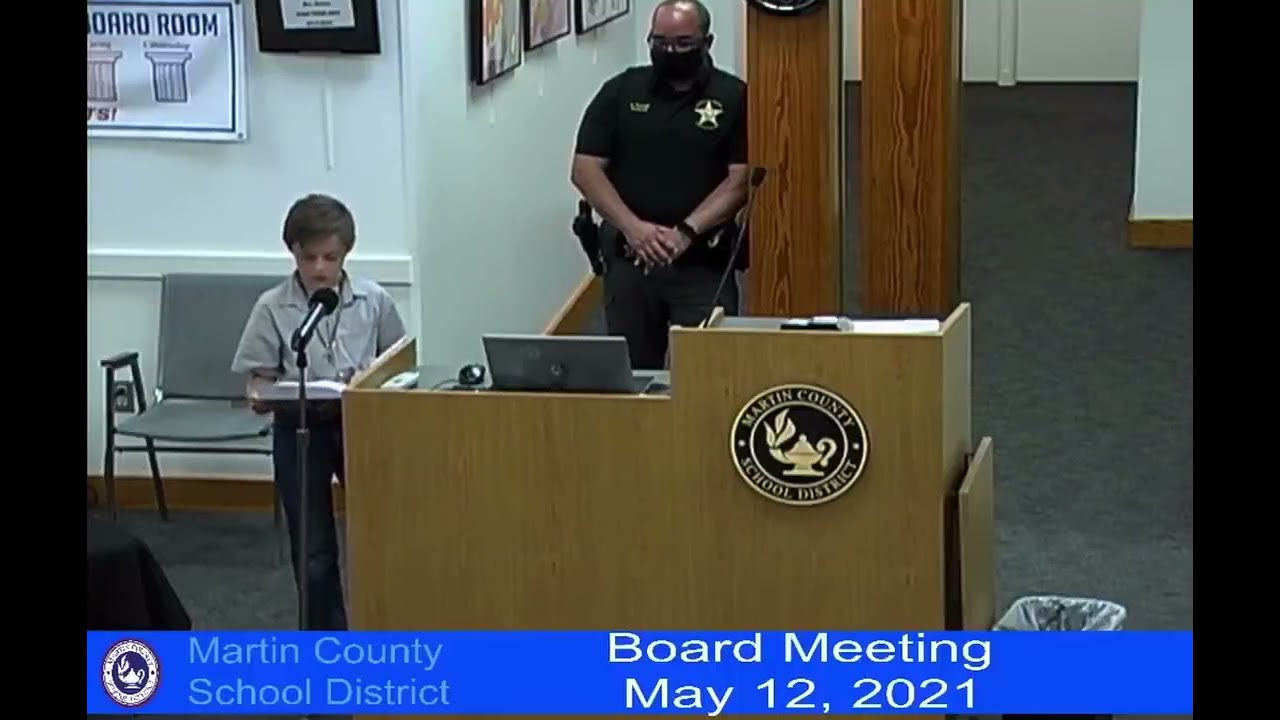In this detailed photograph captured during the Martin County School District board meeting on May 12th, 2021, we see a young boy, likely around fourth or fifth grade, standing at a podium situated to the left of the image. He is addressing the board, speaking into a microphone while glancing down at a piece of paper he holds. The podium bears the Martin County School District seal, a black roundel with white font, and also hosts an open laptop and another microphone.

The boy, with brown hair, is dressed in a white short-sleeve button-up shirt and dark pants. Directly behind him stands a law enforcement officer, identifiable by a star-shaped badge on his left chest. The officer, wearing a black mask, stands with his hands clasped in front of him, leaning against a wooden pillar to his right, with another wooden pillar further to the right.

The setting is a formal, indoor environment typical of a school board meeting, with white walls and a gray chair behind the boy. The lower part of the image features a blue border displaying the text, "Martin County School District Board Meeting May 12 2021," indicating this might be a screen grab from a televised event. The image also includes various other items like signs and framed pictures on the walls, all contributing to the professional atmosphere of the school board meeting. The color palette of the scene is comprised of blue, tan, brown, black, white, gray, and beige.